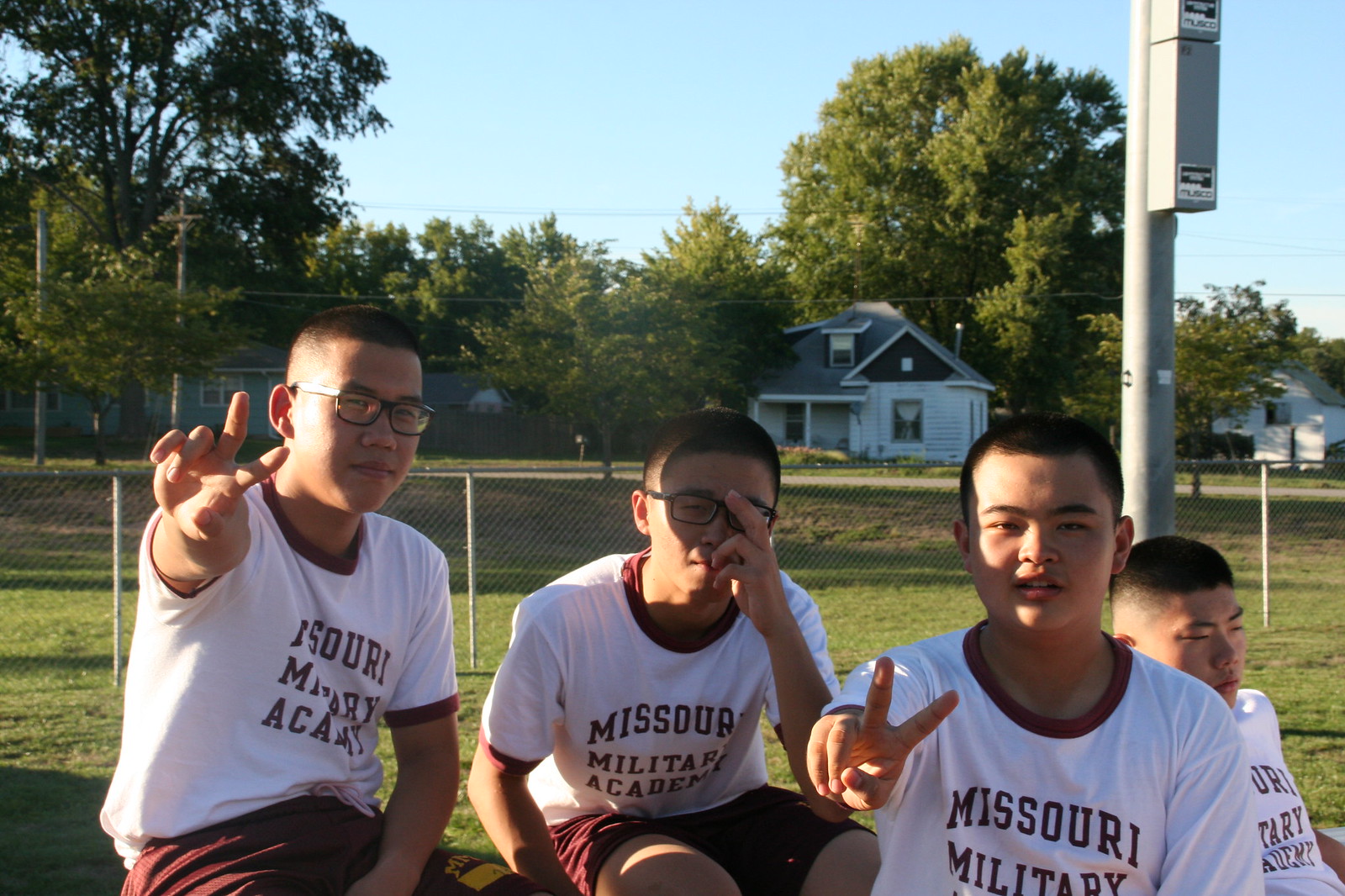This is a detailed photographic image set outdoors during the day, capturing four Asian teenage boys from the Missouri Military Academy. They are all dressed in white T-shirts with red collars and matching red shorts, which display the school's name in red text. All four boys have short, dark brown hair and buzz cuts; two of them are wearing glasses.

The boys are positioned in a row, with two of them giving a V sign with their fingers towards the camera. The first boy and the second boy from the left are both wearing glasses, while the boy on the far right and another next to him are not. The boy on the far right is unique as he is sitting and leaning back, looking away from the camera.

In the background, a rich, green grass field is visible, enclosed by a silver chain-link fence. Further behind, you can spot houses with gabled roofs, some trees, and a clear blue, nearly cloudless sky. A green post and mailboxes are also part of the scene, suggesting a rural neighborhood setting, possibly indicating they are on a break from their military training.